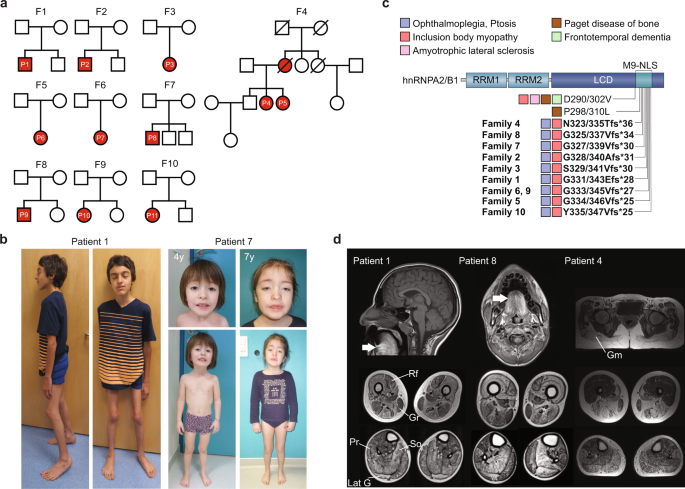This is a detailed and comprehensive image set within a horizontal rectangular layout, comprising four distinct sub-illustrations labeled A, B, C, and D. In the top left, Illustration A features a flow chart resembling a DNA-type chart, interspersed with circles and squares, but devoid of any detailed text except for letters and numbers. Adjacent to it, on the top right, is Illustration C showcasing a variety of microscopic slide images along with a sideways-facing skull diagram. This section also contains relevant information related to the flow chart.

Below the flow chart, in the bottom left (Illustration B), there are thin rectangular photographs depicting two children, identified as different patients at varying stages and ages. Patient one appears as a young boy, while Patient seven is illustrated as a young girl with noticeable changes from ages four to seven.

In the bottom right corner (Illustration D), there are various brain scans and diagnostic images labeled with specific medical conditions such as amyotrophic lateral sclerosis and inclusion body myopathy. This area also includes x-rays for patients one, eight, and four. The entire image is accentuated by a color palette comprising black, white, tan, blue, purple, red, and pink, contributing to the representation of data related to various diseases impacting the children depicted.